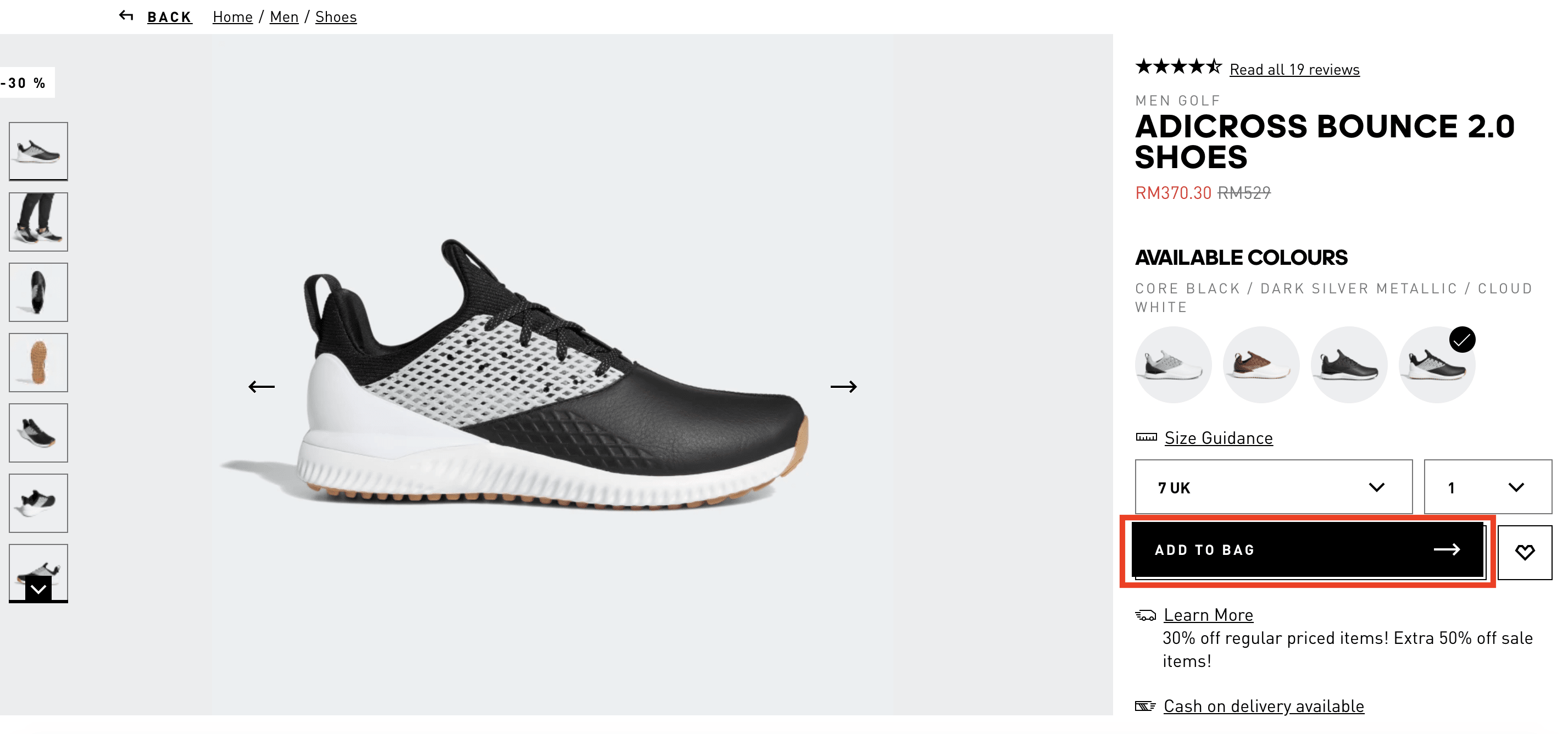In the screenshot of a website, we see a detailed layout centered around a sneaker product. On the left side, within a light gray box, there's a prominent image of a sneaker – specifically, the left shoe in a profile view – displayed in black and white. This main image is accompanied by a series of smaller thumbnails beneath it, showcasing different angles and details of the shoe.

Above this section, a navigation menu is presented in black text, listing options for 'Back,' 'Home,' 'Men,' and 'Shoes.' To the right of the sneaker image, set against a white background, there is a rating indicator displaying four and a half black stars. Accompanying the rating is a link in black text inviting viewers to "Read all 19 reviews."

Directly below, in bold black large text, the product name is highlighted: "AD Across Bounce 2.0 Shoes." Further down, in smaller text, the available colors for the shoe are listed as "Core Black/Dark Silver Metallic/Cloud White."